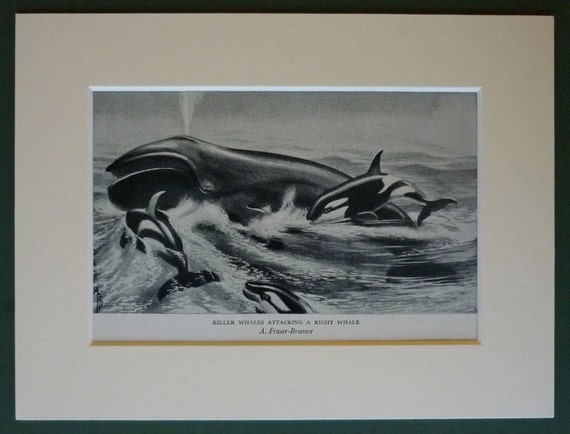The image depicts a framed, old-style black and white naturalist etching titled "Killer Whales Attacking a White Whale." The artwork, likely crafted around the turn of the century, shows a dramatic maritime scene. At the center of the action, a white whale surfaces, expelling water from its blowhole amidst a tumultuous sea. Surrounding it are three killer whales; one leaps exuberantly to the right, another rides a wake on the left, and the third lifts its head just above the image's border, creating swirling wakes all around. The hazy, cloudy sky looms in the background, contributing to the tense atmosphere. The piece is framed in a simple black frame with thick tan matting, bevel cut to reveal a white interior edge. Though the artist's name in italic is not fully legible, the etching bears a stark and heavily shaded aesthetic reminiscent of classic book illustrations.